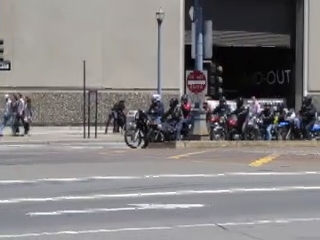In this slightly grainy, low-resolution daytime photograph, we capture an urban scene dominated by a large gray and tan building. Only the base of this flat-surfaced building is visible. The focal point of the image is a group of nearly 12 or 13 motorcyclists, all wearing helmets, who are lined up horizontally from the center toward the right side of the frame. They appear to be waiting, possibly at a traffic light or preparing to start their ride. Directly behind them, a sidewalk is visible, dotted with pedestrians casually walking by. The multi-lane road they are on features three distinct horizontal white painted lines, indicating the lanes. The bikers are positioned just behind a signpost, which supports a street light and a slightly blurred white sign that seems to read "Do Not Enter."